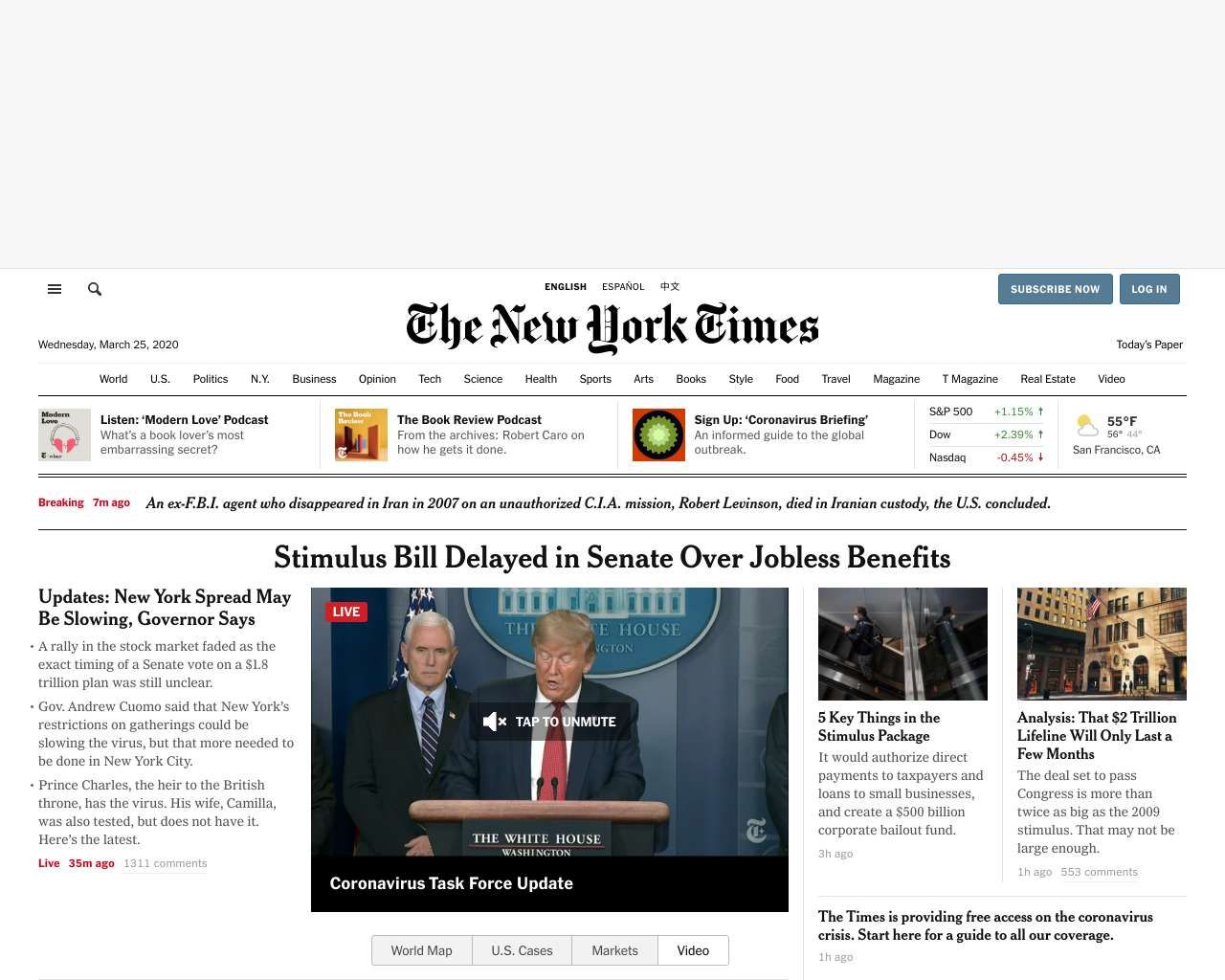This image is a screenshot of the New York Times homepage, oriented in landscape. The layout features a gray rectangle across the top of the screen without content, followed by a white rectangle with the newspaper’s headline.

At the very top, in small font, there is a hamburger menu and a search bar. To the top right are two blue rectangular buttons: "Subscribe Now" and "Login."

Centered at the top is the iconic "The New York Times" logo, accompanied by the date, "Wednesday, March 25, 2020." Just below this, navigation options categorize articles into sections such as World, U.S., Politics, New York, and Business.

The main section is bordered and contains various article links and multimedia elements, including a prompt to listen to the Modern Love podcast, the Book Review podcast, and a link to sign up for Coronavirus briefings. It also displays stock prices and the current weather for San Francisco.

A breaking news header from seven minutes ago introduces the main headline: "Stimulus Bill Delayed in Senate Over Jobless Benefits," accompanied by a thumbnail image of Donald Trump and Michael Pence. Other articles are listed beside the main headline, forming a comprehensive and detailed snapshot of the day’s significant news.